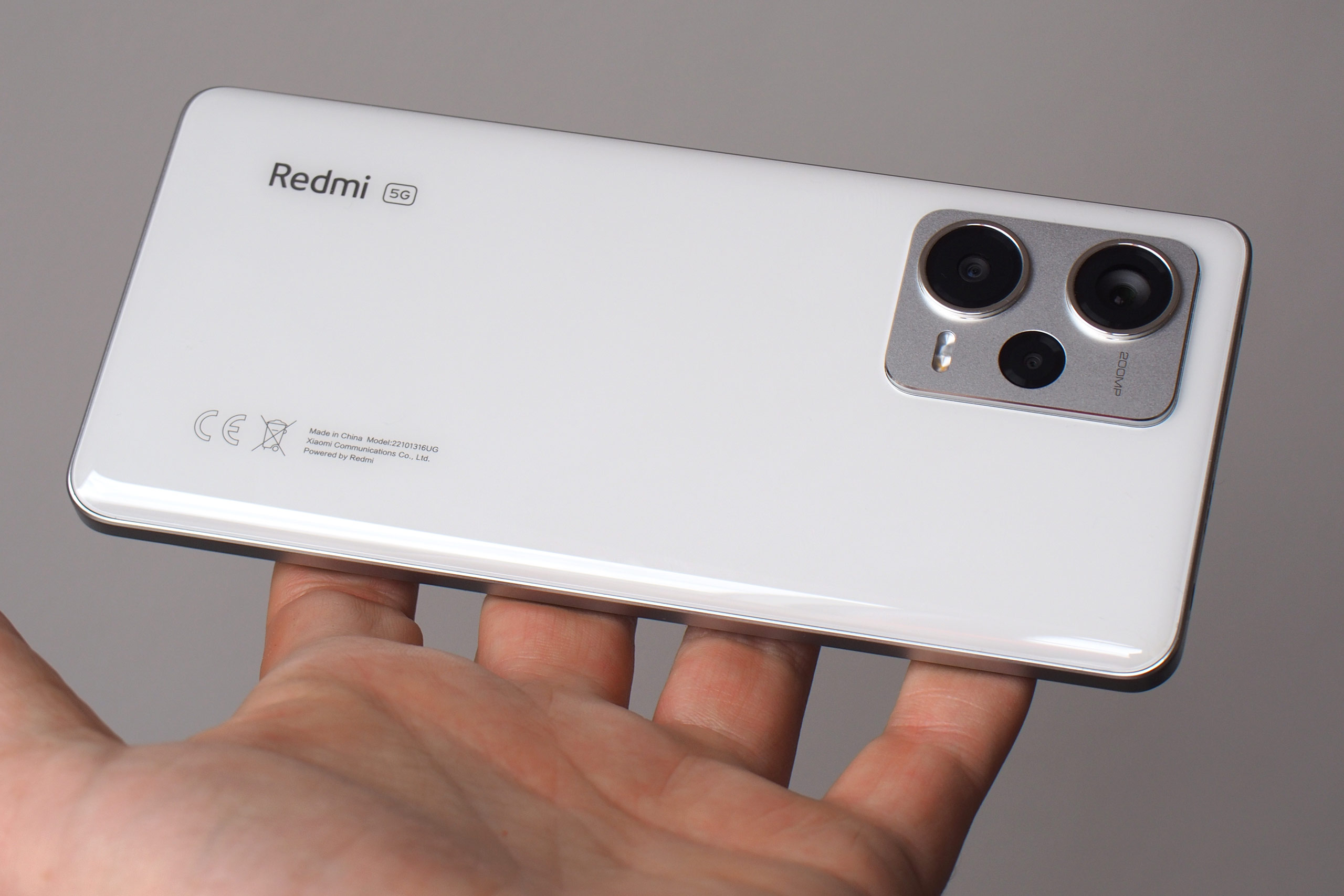In this detailed color photograph, the subject is a white Redmi 5G smartphone. The image is captured in landscape orientation from a top-down perspective, with a beige-brown background. A person's hand, visible from the palm side with fingers extended and slightly spaced apart, holds the phone horizontally at the fingertips. The phone, which appears extremely thin, has a silver edge around it and a silver camera frame in the top right corner. On this frame, there are three lenses positioned vertically—two large ones and a smaller lens beneath them, along with what seems to be an LED flash. Engraved on the camera frame, it says "200 MP," indicating the camera's resolution. On the top left corner of the phone, there is black text that reads "Redmi" followed by "5G" in a small rectangle. Near the bottom left corner, additional small black text features technical notations indicating manufacturing details, including "Made in China Exmoe Communications powered by Redmi," alongside an icon of a garbage can with an X through it. The overall style of the photograph is representational realism.